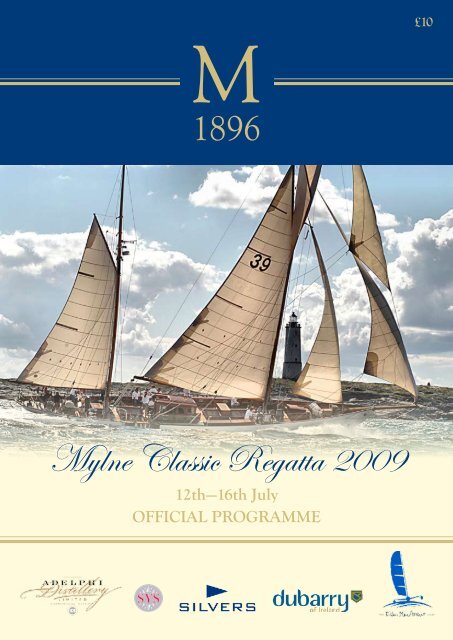The image depicts the cover of the official program for the Milne Classic Regatta, held from the 12th to the 16th of July in 2009. The design predominantly features navy blue, gold, and white colors. At the center is a striking photograph of a large sailing ship with multiple sails, five to six on two masts, with the number 39 prominently displayed on one of the sails. The ship, which appears to carry around 11 crew members, is tilted to the side as it navigates through choppy seas. In the background, there's a scenic view of land with a lighthouse, set against a sky filled with fluffy clouds. Above the photograph, centered on the page, are the letter "M" and the number "1896". The upper right corner bears the price of 10 pounds. Below the photograph, the text reads "Milne Classic Regatta 2009 12th to 16th of July official program," accompanied by sponsor logos for companies such as SVS, Dubarry, and Silvers at the bottom part of the frame.